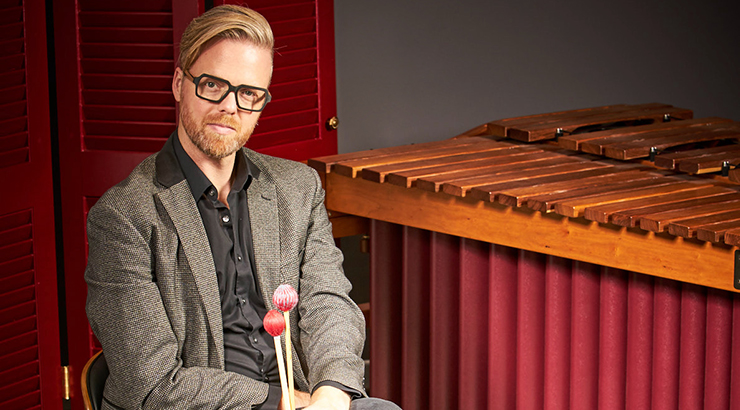In the image, there is a man sitting confidently in a chair, donning a gray suit jacket over a black button-up collared shirt. His top couple of buttons are casually unbuttoned. He wears black glasses, and his blonde hair is slicked back or combed to one side, complementing his light scruffy beard and mustache. His expression is proud and inviting, as if he's ready to perform.

Next to him stands a large wooden xylophone or marimba. The instrument is quite striking with its polished wooden bars and rests on a stand draped with a red cloth. He holds two xylophone mallets, characterized by their wooden handles capped with round red tips. Above and behind him is a red folding door, resembling a Japanese-style shutter or accordion partition with a little golden knob. The background is a subdued gray, which contrasts with the red elements and draws attention to the man and his musical setup. The overall setting exudes a poised yet inviting atmosphere, as if the man is ready to play the instrument and engage with the viewer.